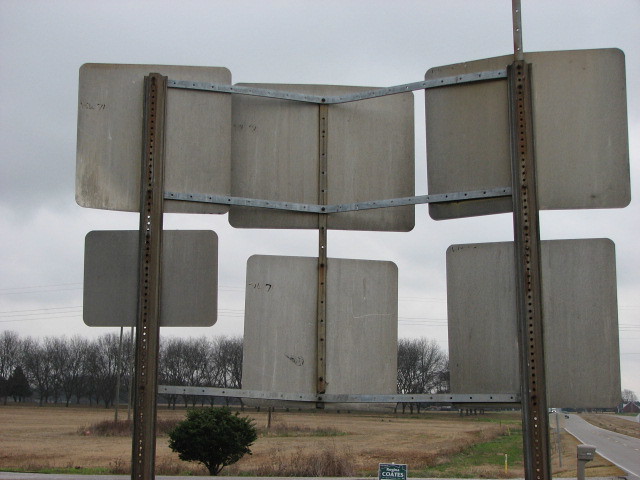The photo captures a dreary scene on what appears to be a late fall or winter day, characterized by overcast skies and a general gray gloom. The main focus is on the backside of six street signs mounted on two vertical metal posts, with additional beams connecting them for stability. The surrounding landscape features a mix of brown and dead patches of grass, giving a sense of the season. In the background, there's a row of leafless trees and a field. The right side of the image reveals a road or highway, where you can spot a car in one of the lanes, its headlights visible, and electrical poles carrying lines above. A small mailbox and a picket sign stating "coats" add minor details to the otherwise muted scene.